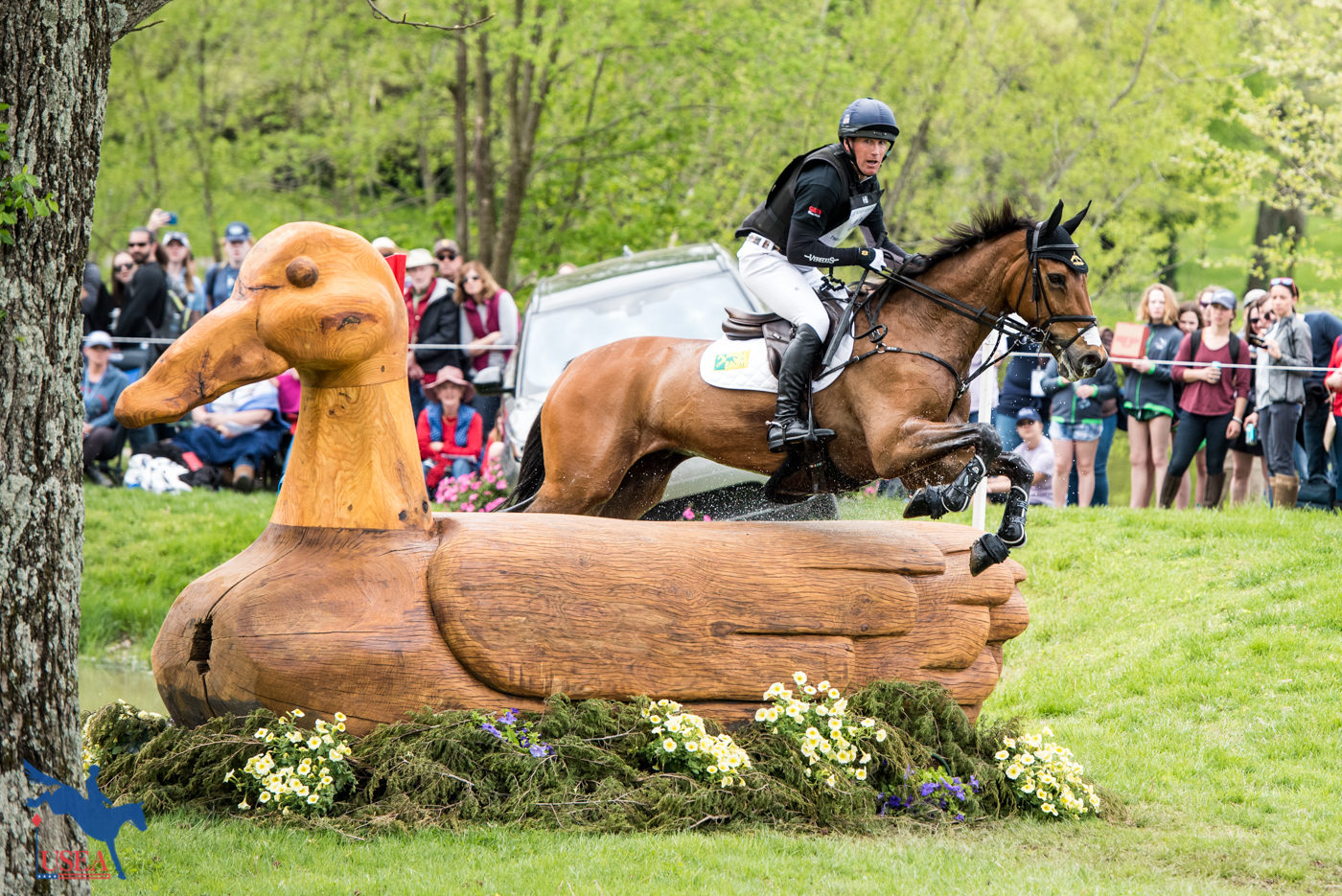In this outdoor scene set in a lush, green environment with numerous trees in the background, a dramatic moment unfolds as a jockey on a brown horse with a black mane and tail leaps over a large wooden duck obstacle. The horse, bearing a white spot above its nose, is captured mid-air, with water splashing around them. The rider is outfitted in a black helmet, a black long-sleeved shirt with a red logo on the side, blue pants, and black riding shoes. Surrounding the wooden duck, which has a lighter wood head and neck and a darker wood base, are ferns and flowers. People stand behind a rope barrier, watching the event unfold with a large tree trunk visible on the far left, extending to a backdrop filled with more trees. The area features a grassy riding path and a green slope leading up to where the bystanders are gathered.